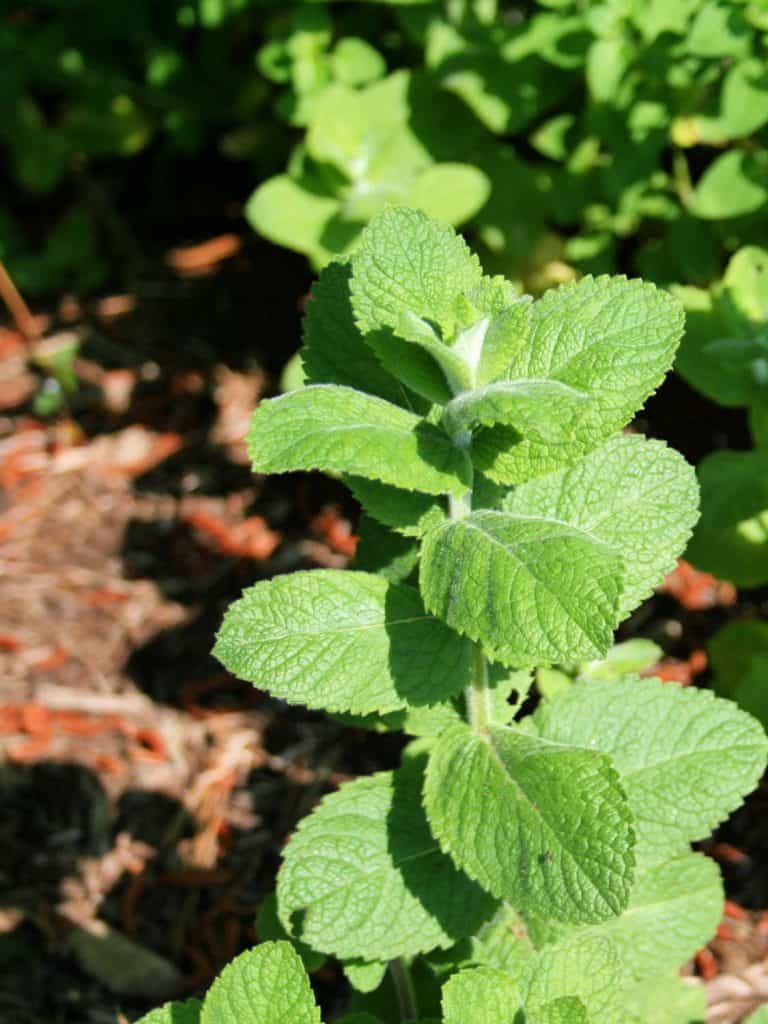The image is a detailed close-up of a mint-like plant, potentially an apple mint, prominently situated in the center of the frame. The plant's vibrant green leaves, numerous and of similar size, are characterized by jagged, sawtooth edges and a rugged texture. Each leaf displays a central tan-colored spine that supports its structure. Some leaves exhibit slight sun damage, with their edges tinged tan, but overall, they maintain a healthy green hue. The leaves alternate along the stem, which adds to the plant's visual interest. The background is out of focus, revealing numerous similar plants, giving the impression of a dense, green garden. The ground beneath features brown and slightly reddish wood chips, adding a contrasting layer to the green foliage. The upper left corner of the image is notably darker, likely due to shadows, while the right-hand corners are blurred, suggesting the continuation of more plants.